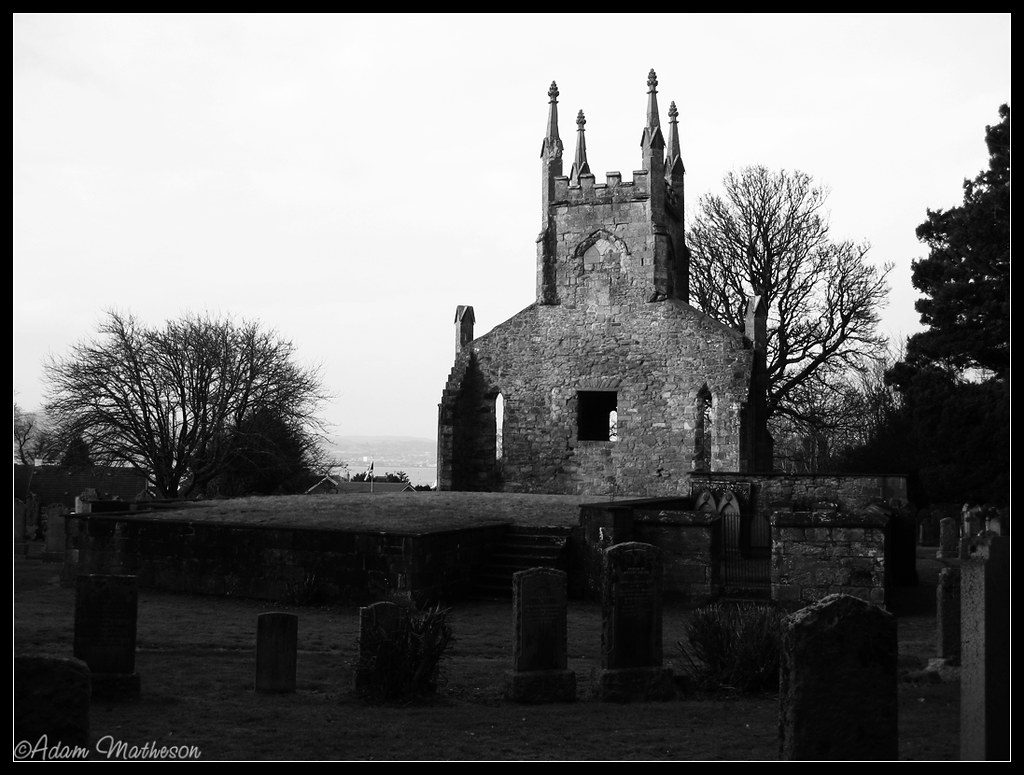The black-and-white photograph, attributed to Adam Matheson with copyright visible in the lower right-hand corner, captures an eerie and timeless scene. The central focus is an ancient stone structure, which appears to be either a small castle or a chapel, distinguished by its four spires and intricate stone inlay. This structure seems to be in some state of ruin, suggesting it may once have served as a church. In the background, a bright, white sky contrasts with leafless trees, indicative of the winter season, except for a solitary evergreen tree on the right. The foreground is populated with withered and aged gravestones, clustered together, evoking the sense of a historic cemetery. Two bushes break the monotony of the grave markers; one is centrally located while the other is towards the right. Further details in the photograph include a set of stairs leading to a platform in front of the stone structure, and a single window piercing its facade, enhancing its aged and mysterious character.